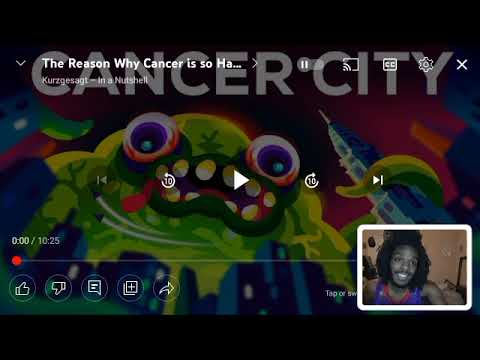The image depicts what appears to be a screenshot of a YouTube video titled "The Reason Why Cancer is So HA..." Above this title, in large light gray capital letters, are the words "Cancer City." The video thumbnail showcases a cartoon- or computer-generated roundish green monster with big round eyes and a gaping mouth full of sharp white teeth. The monster has tentacle-like arms, with one arm wrapped around a large building, suggesting a backdrop of tall city buildings. The image has black borders on the top and bottom.

Below the thumbnail, there is a progress bar indicating the video is 10 minutes and 25 seconds long, showing "000/1025" with a red dot at the left. Next to this bar are five circular icons including thumbs up, thumbs down, a text box, and an arrow. In the bottom right corner of the image, within a white-bordered box, is a video connection window featuring a smiling black man with dreadlocks, dressed in overalls. He appears to be preparing to react to the video.